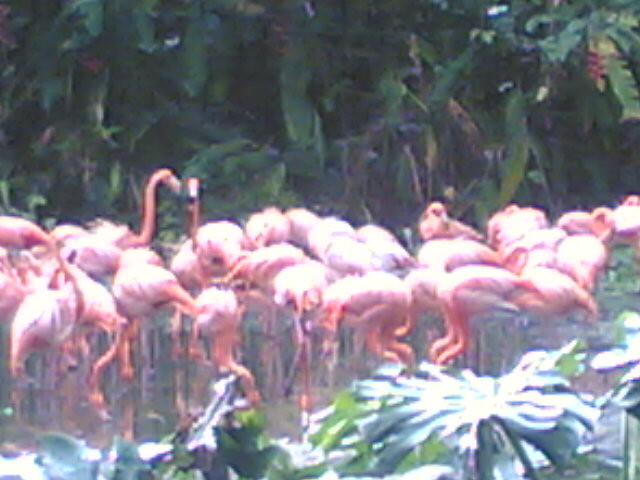The photograph captures a flock of pink flamingos standing and foraging in a shallow pond, surrounded by lush, tropical vegetation. The image, which appears to be somewhat pixelated and grainy, suggests it might be a screenshot or video capture. In the center of the picture, around 25 to 35 flamingos are grouped together. Most have their heads submerged in the water, likely searching for food, while a few have their heads raised, looking around. The scene is framed by sunlit tropical leaves in the foreground, and behind the flamingos, a dense backdrop of palms, moss-covered trees, and other vibrant green foliage creates a picturesque setting. Despite the blurriness, the contrast between the pink of the flamingos and the rich greens of the surroundings is striking.